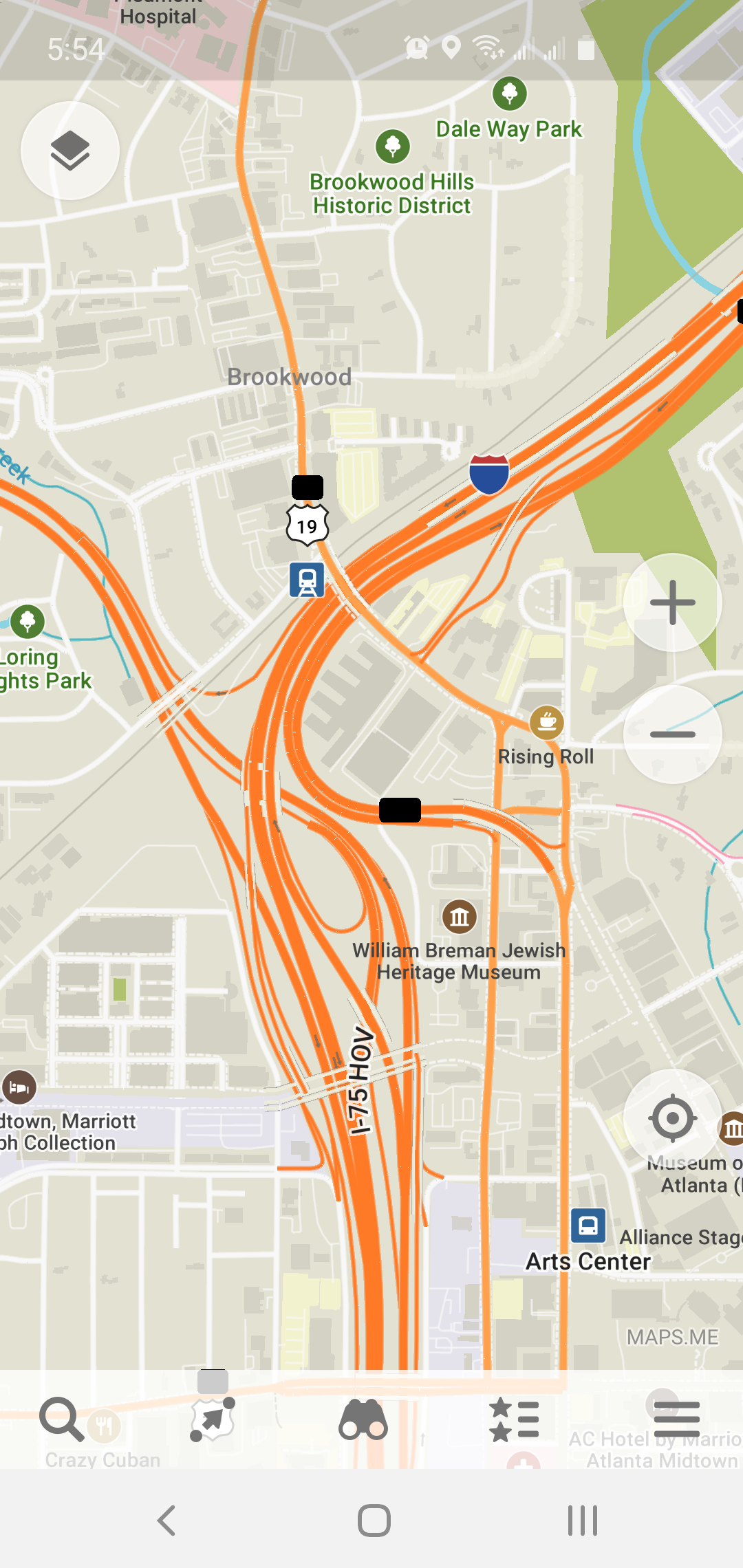The image is a vertically oriented screenshot of a cell phone display, approximately two to three times taller than it is wide. At the top of the screen, the time "5:54" is displayed in white on the upper left, with six status icons, including wireless signal strength and battery life, aligned slightly indented from the upper right.

Below the status indicators, the main content of the screenshot is a map, likely from an app such as Google Maps or a similar service. The map prominently displays several highways, rendered in orange, beginning at the bottom of the screen and curving upwards and towards the right in a roughly 130-degree direction until they extend off the screen. Key locations are marked on the map, including "Art Center" at the lower right, "Brookwood Hills Historic District" at the top, and "Dale Way Park" situated nearby. The major road "I-75 HOV" is also highlighted in orange, indicating its significance in the area.

At the bottom of the screen, there are five icons for navigating within the app and the standard navigation buttons typical of a cell phone interface.